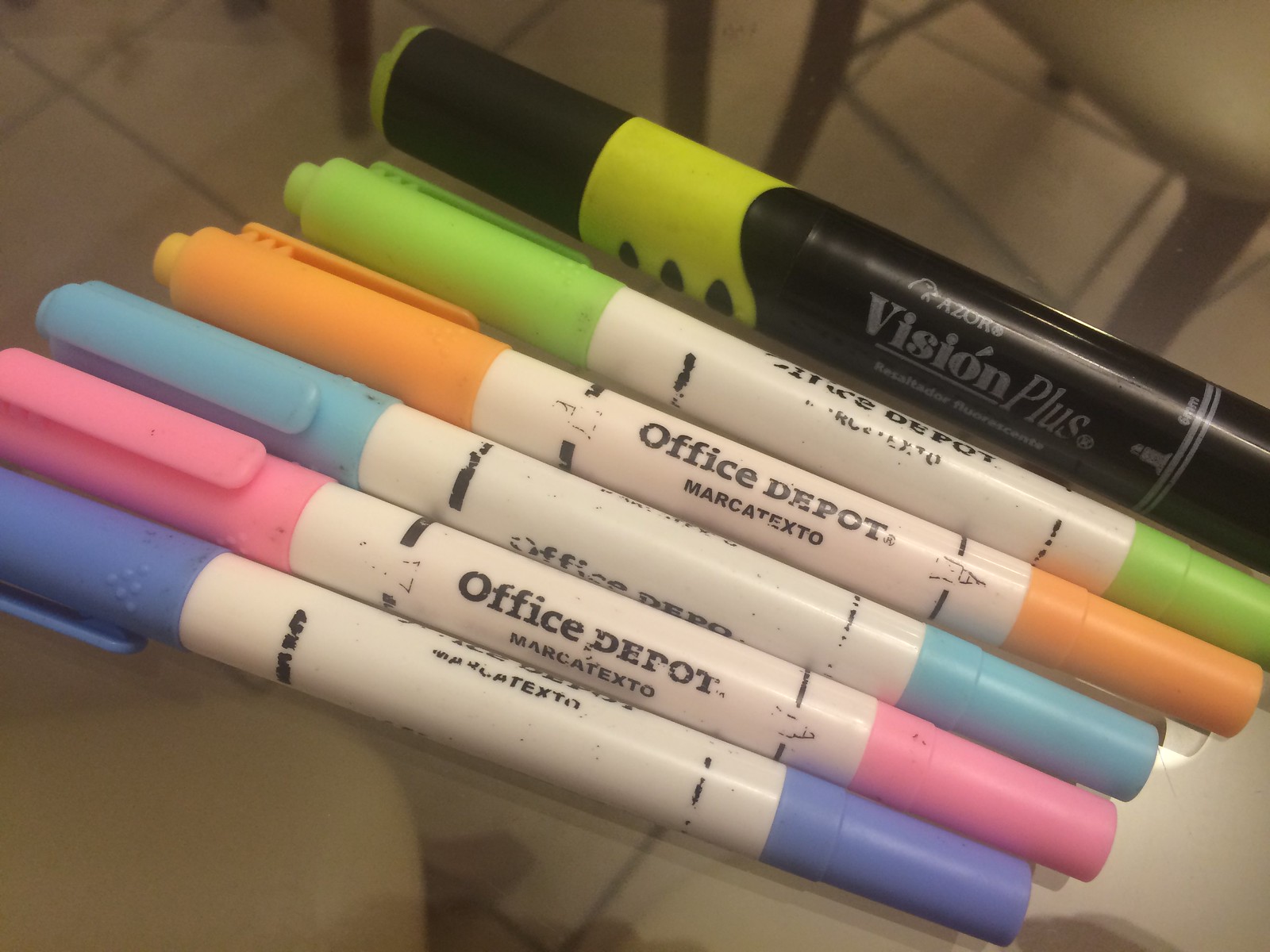The image depicts a row of distinctly colored markers neatly arranged on a glass table, through which is visible a white-tiled floor and part of a brown wooden chair with a white upholstered seat, hinting at a dining area setting. There are six markers in total: five of them feature a white base with black "Home Depot" lettering, paired with vivid caps on either end—bright green, orange, light blue, pink, and a darker blue. The print on these markers is somewhat worn. The sixth marker, contrasting with the others, is a Vision Plus marker, notable for its black body and fluorescent yellow highlights, resembling a large highlighter. The markers are positioned horizontally and closely lined up, contributing to a visually organized and colorful display.